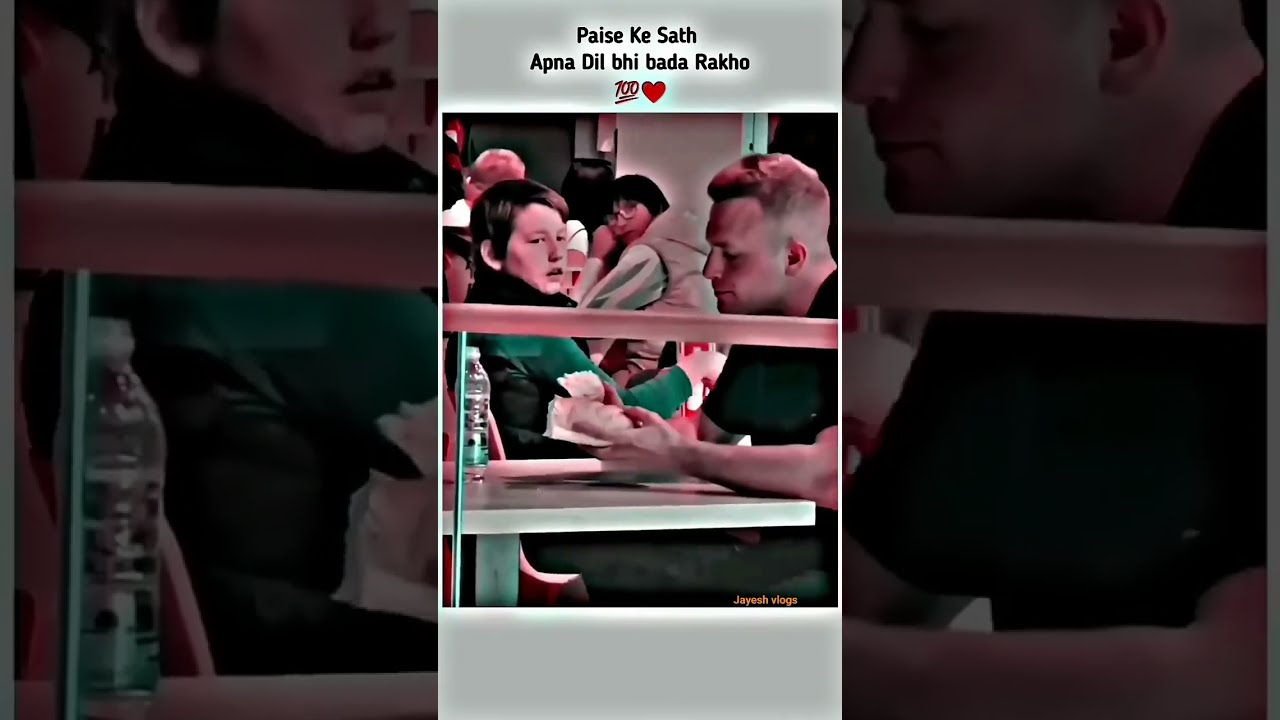The image is a horizontally rectangular photograph divided into three sections: left, center, and right. The left and right sections are from the same picture, but darker, and show close-ups of two individuals seated at a table. The middle section, which is lighter and superimposed over the left and right, includes the entire picture. In this section, there are two main individuals in the foreground. The person on the left is looking forward and slightly to the right, wearing a dark jacket with green sleeves. On their right forearm lies a wooden railing, and a water bottle sits on the table in front of them. The person on the right has short hair with sunglasses on top of their head, a dark and green-colored shirt, and is resting their arms on the table, looking to the left. The background shows other seated individuals, including a woman with black hair and glasses resting her face on her hands. Text in black, non-English font appears at the top of the middle section within a gray rectangle, alongside a red heart symbol and another red heart below. The left image is a close-up of the left person, cut off at the nose and distinctly showing the water bottle and railing. The right image is a close-up of the right person, cut off above the eyes, easily showing the railing and their left arm down to the wrist. All sections of the image depict an indoor setting, capturing a group of people seated around a table.